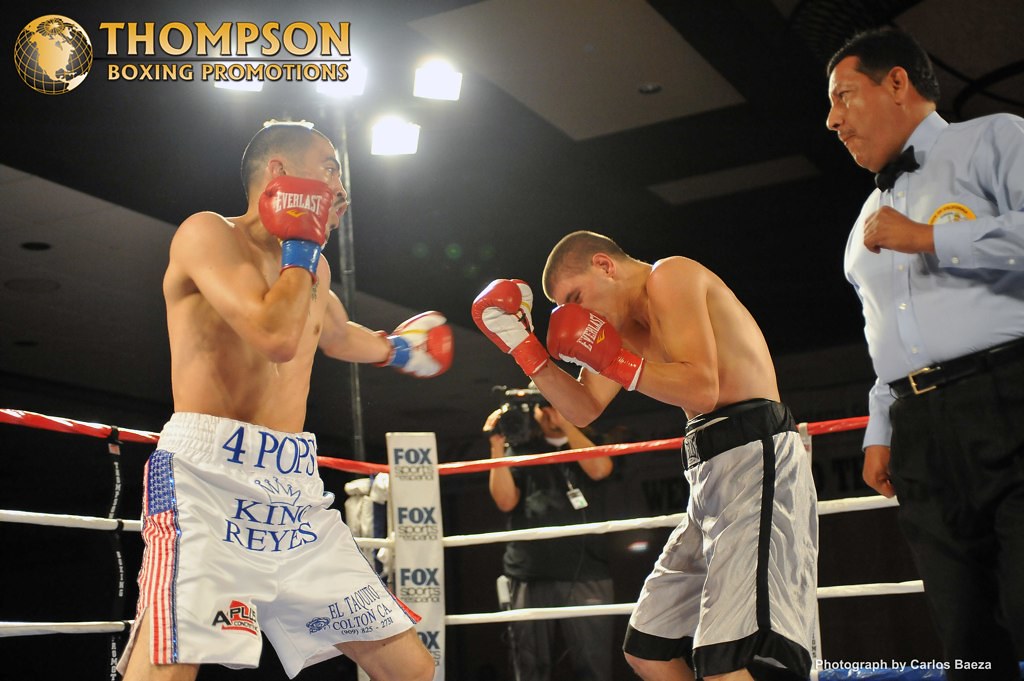The image captures an intense moment in a boxing ring under the banner of Thompson Boxing Promotions, with its gold lettering and accompanying gold continent globe positioned in the upper left corner. The two boxers, both wearing red gloves, are in the midst of a punch exchange. The boxer on the left, dressed in white shorts adorned with "Four Pops," "King Reyes," and an American flag, is delivering a punch. His opponent, in gray trunks with black stripes, is ducking to avoid the hit. A referee, positioned slightly behind and to the right, is dressed in a blue shirt with a yellow emblem, a black tie, black pants, and a black belt, seemingly moving around the fighters. The red and white ring ropes frame the action while the spotlights overhead illuminate the dark ceiling, highlighting the intensity in the ring. Additionally, a "Fox Sports" logo is visible on one of the ring posts, and a cameraman is stationed outside the ring, capturing the match.